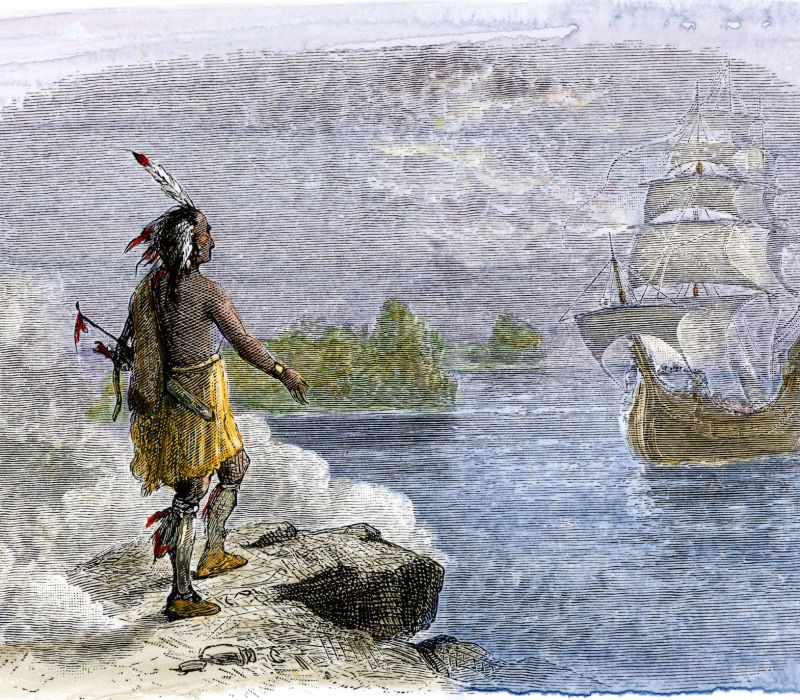In this historic hand-drawn illustration, a Native American man is depicted sitting on rocks by the water, looking towards a distant boat with four large white sails on a blue, smoky horizon. The detailed figure, shirtless, is adorned with distinct yellow attire—a skirt, shoes, and a scarf draped over his shoulder. He also wears white stockings and has a red band tied around his leg. His head is decorated with a collection of feathers, white and pink, as well as black-tipped ones. A watch is visible on his outstretched arm, and he carries weapons on his back. The scene portrays a moment of contemplation as he gazes at the boat, possibly witnessing it for the first time, against the backdrop of green trees and a white sky.